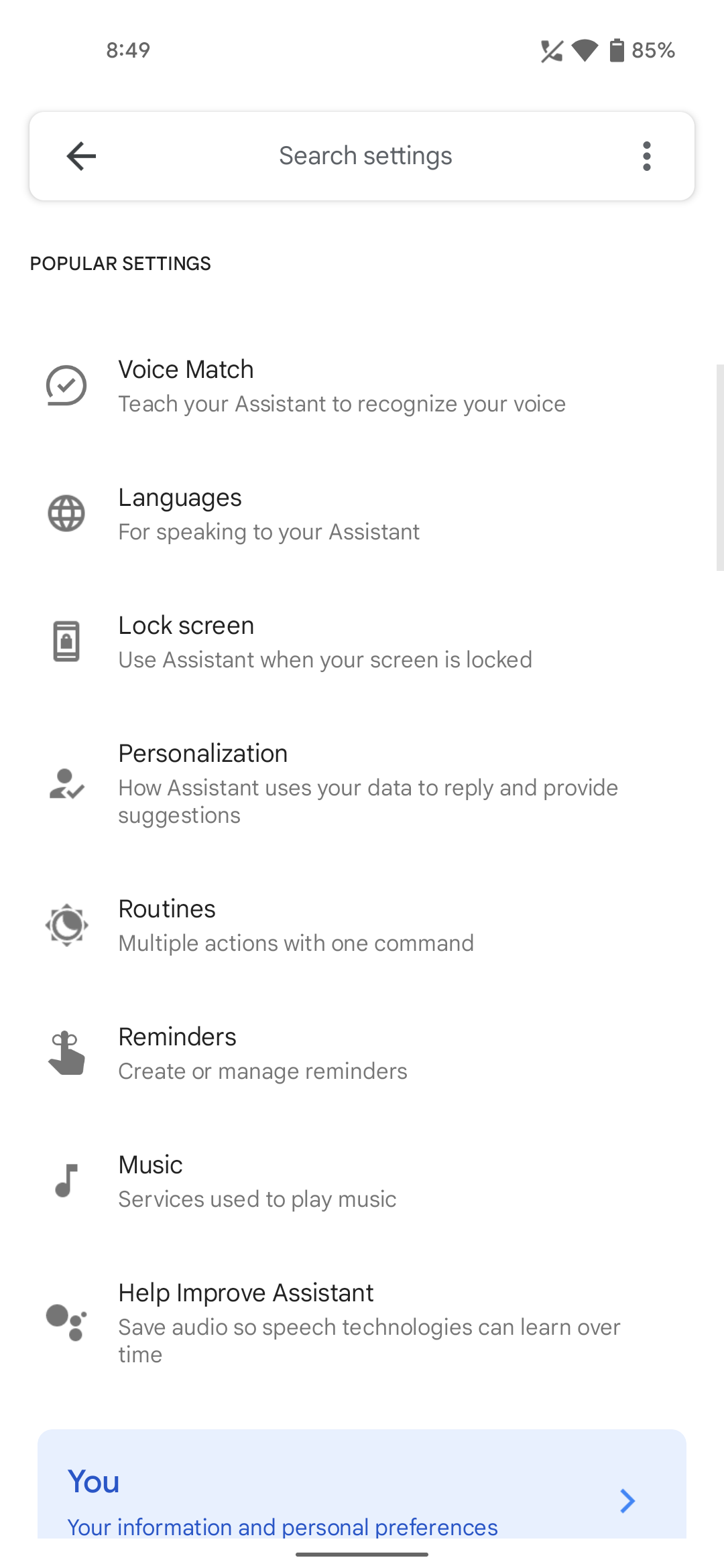This detailed image showcases a smartphone screenshot displaying personalization settings for the lock screen and voice match features, among others. The screenshot reveals the time as 8:49 AM, found at the top of the screen. The status bar shows a phone receiver icon with a slash through it (indicating Do Not Disturb mode), a full Wi-Fi signal, a vertically-oriented battery icon labeled with 85% power remaining, a back arrow, a magnifying glass for search settings, and three vertical dots, indicative of additional options, positioned on the right.

The main section of the screenshot features the popular settings for a voice assistant, possibly Google Assistant, totaling eight distinct options, each accompanied by a simple gray icon:

1. **Voice Match (Circle with a check mark)**: Allows you to teach your assistant to recognize your voice.
2. **Languages (Globe)**: Pertains to the languages used for communicating with your assistant.
3. **Lock Screen (Smartphone)**: Provides the option to use the assistant even when the screen is locked.
4. **Personalization (Person with a check mark)**: Explains how the assistant utilizes your data to offer responses and suggestions.
5. **Routines (Sun with a moon inside)**: Enables the execution of multiple actions with a single command.
6. **Reminders (Hand with a bow-tied finger)**: Allows you to create and manage reminders.
7. **Music (Musical note)**: Refers to the music services used for playback.
8. **Help Improve Assistant (Assistant logo with four dots)**: Saves audio so speech technologies can improve over time.

At the bottom of the screen, there is a blue-highlighted option labeled "You," which likely leads to a section detailing personal preferences. This label sits alongside a right-pointing arrow, suggesting further navigation options.